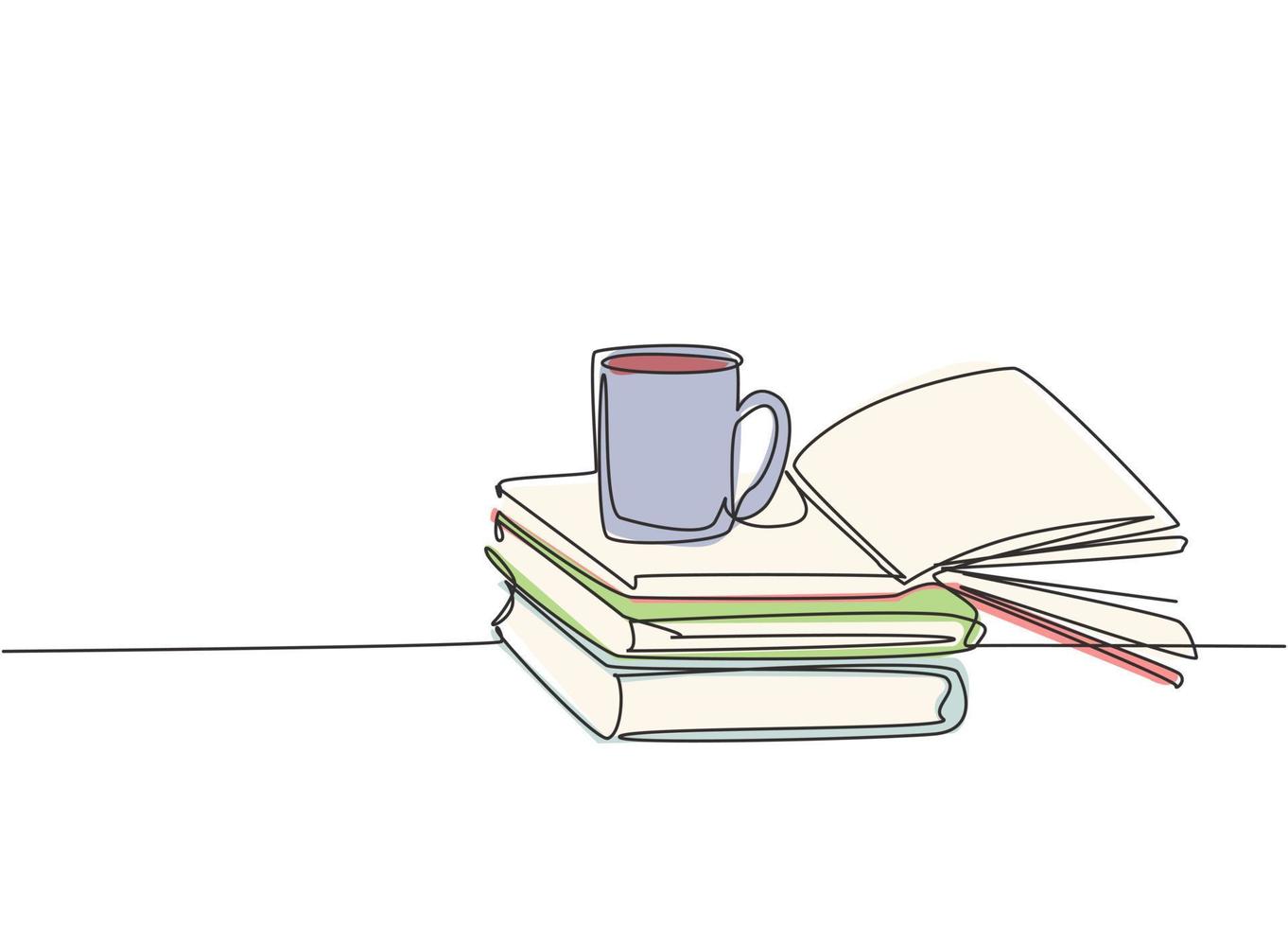The image features a simplistic yet detailed sketch of three stacked books and a coffee cup on a table, all created with a continuous line style that evokes a mid-century artistic vibe. Starting from the bottom, the stack includes a closed blue book, followed by a light green book, and a red book on top that is halfway open. The open red book has its pages slightly fanned out over the edge of the table, with no text on the blank white pages. Resting within the folds of the open red book's pages is a light purple coffee mug containing a red liquid, possibly coffee or tea. The table is indicated by a single horizontal line, adding to the minimalist charm of the entire drawing. The simplicity in the illustration captures a moment of study or leisure frozen in time.